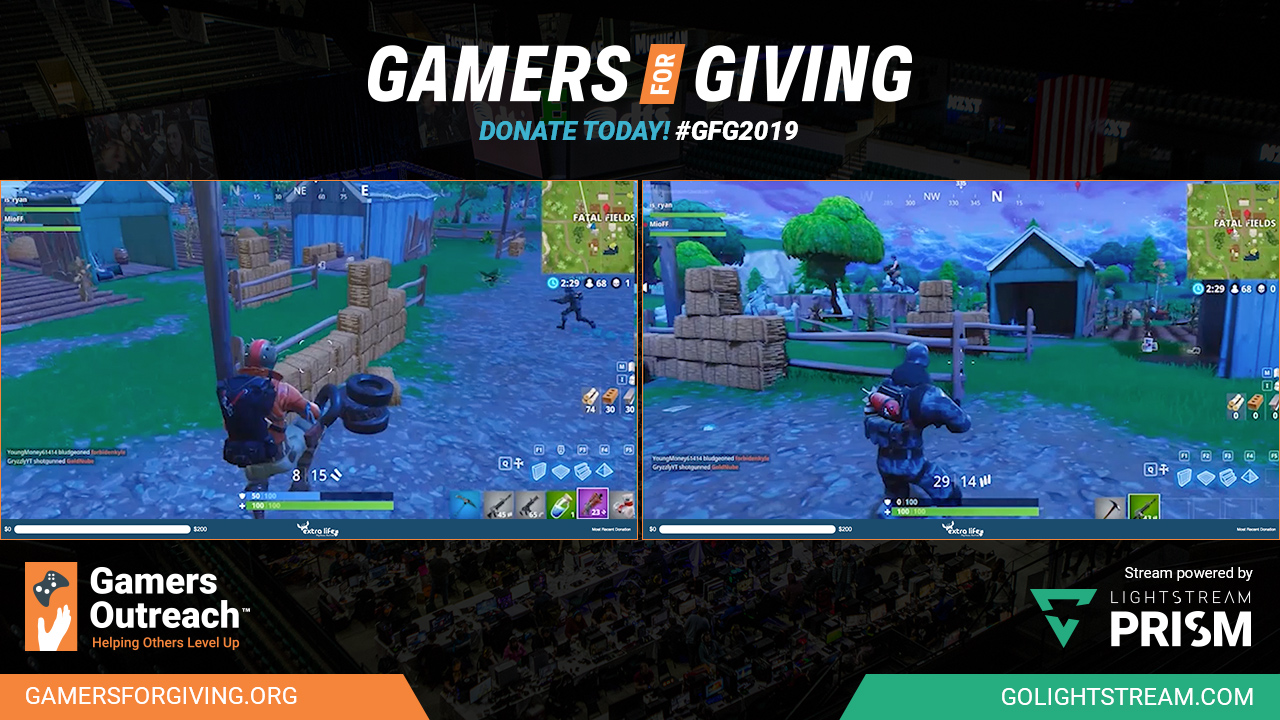This image features a detailed advertisement from a gaming charity event known as "Gamers Forgiving 2019." At the top of the image, the event's title "Gamers Forgiving" is displayed in bold white text, accompanied by the call to action "Donate Today" in blue, and the hashtag #GFG2019. The text is set against an orange background with white text.

The image showcases two screenshots from a shooter video game. In each game scene, there is a character. The character on the left is dressed in an orange outfit with a black backpack, while the character on the right is in an all-blue outfit with a backpack as well. Both scenes depict nature settings with hay bales, trees, and buildings. Characters appear to be actively engaged, possibly aiming or running, with other figures visible in the background. A map is positioned at the top right of both screenshots.

At the bottom left, the text reads "Gamers Outreach: Helping Others Level Up, gamersforgiving.org," while the bottom right corner states, "Stream powered by Lightstream Prism, golightstream.com." The advertisement combines visual elements of the game with promotional material for the charitable cause.